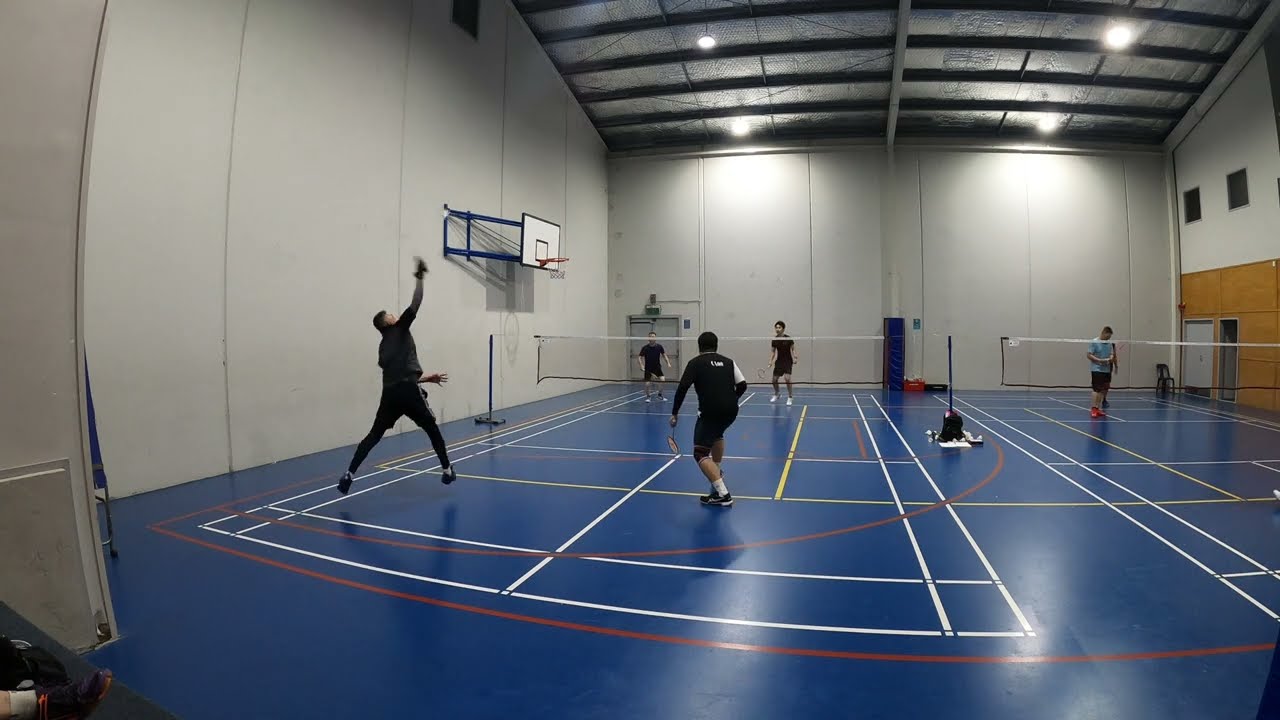The image depicts an indoor gymnasium with two adjacent blue badminton courts featuring yellow, white, and red stripes. The gym walls are predominantly gray, and the ceiling is high with lights. The court on the left is fully visible, hosting a doubles badminton match with four players dressed in black, one of whom is jumping to hit a shuttlecock, while the others focus on the game. On the right court, slightly obscured on the lower right, a single player wearing a light blue shirt and black shorts stands ready behind the net. The gym also features a basketball hoop and a white door with a wooden bottom half on the right side.